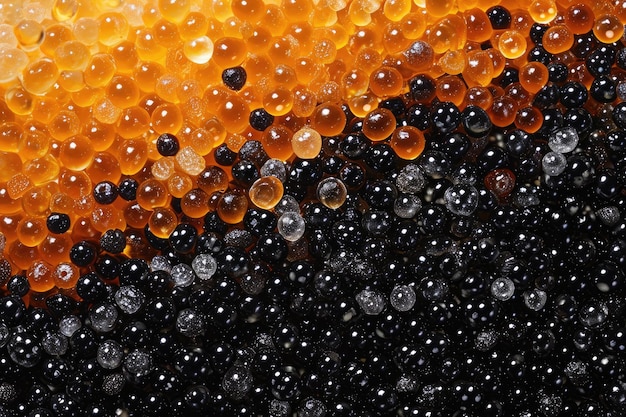This is an extreme close-up photograph showcasing two types of caviar. The upper left corner of the image features small, translucent orange fish eggs that lighten towards the top and gradually transition into a richer, yellowish-orange hue as they move diagonally downward to the center. These orange eggs then blend into darker hues and become black caviar, occupying the bottom right half of the frame. Each egg appears smooth, polished, and wet, reflecting light as tiny white dots. The orange and black eggs intermingle where they meet, creating a gradation of colors. The image captures the intricate details and texture of over 200-300 tightly grouped eggs, presenting a visually organized and striking pattern.